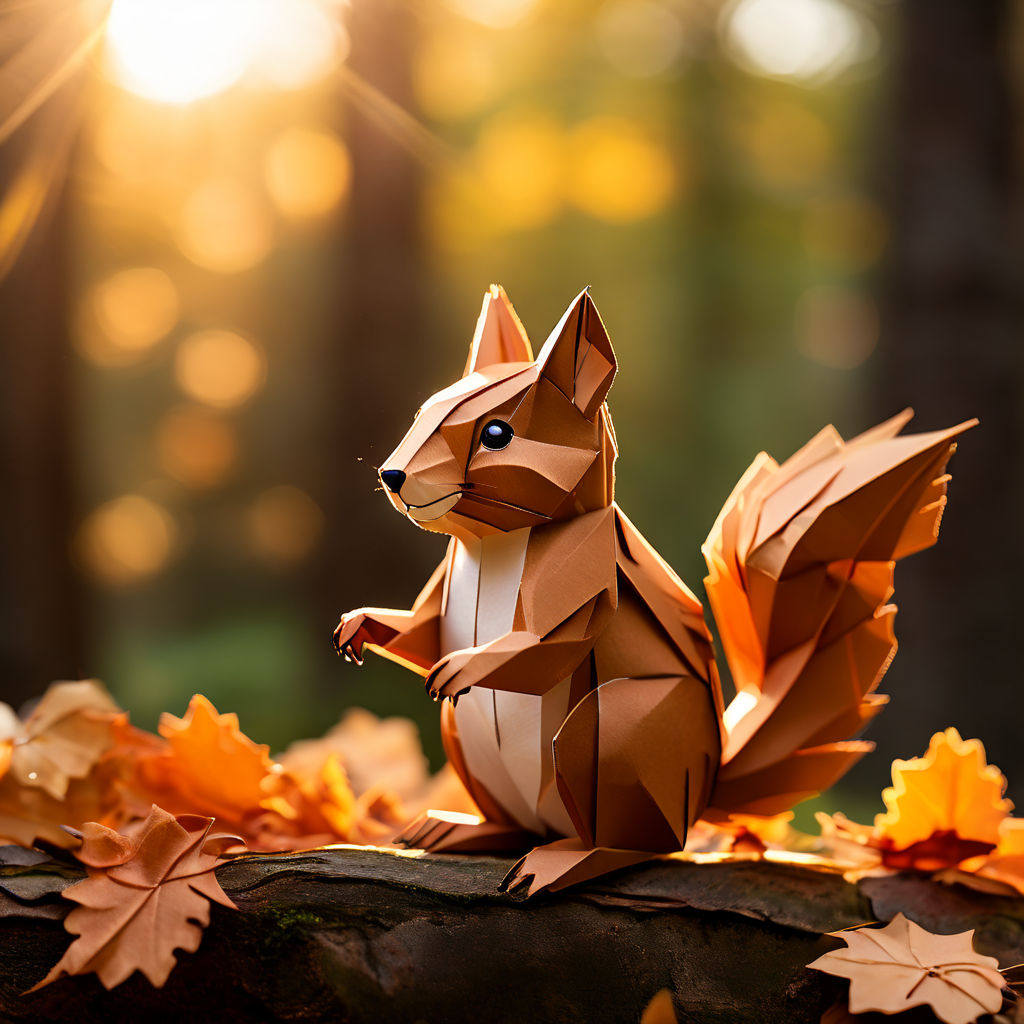In this mesmerizing image, the central figure is an intricately crafted origami squirrel, showcased amidst a blur of amber, tan, and dark brown hues in the background, hinting at a sunlit forest. The detailed craftsmanship captures every aspect of the squirrel, from its brown-tipped nose to its expressive dark brown eye and white chest area. This impressive paper sculpture features a bushy, fluffy-looking tail in shades of brown and amber-orange, poised diagonally with the tail flaring upwards to the right.

The squirrel is perched seamlessly on what appears to be a wooden log or branch, with two of its feet planted firmly while the other two extend ahead of it. This log is enveloped by fall-colored leaves on both sides, which may also be crafted from paper or felt, adding to the cohesive artistic composition. The backdrop, though blurred, suggests a serene forest bathed in sunlight, illuminating this extraordinary piece of paper art that stands out in its lifelike precision and geometric perfection.